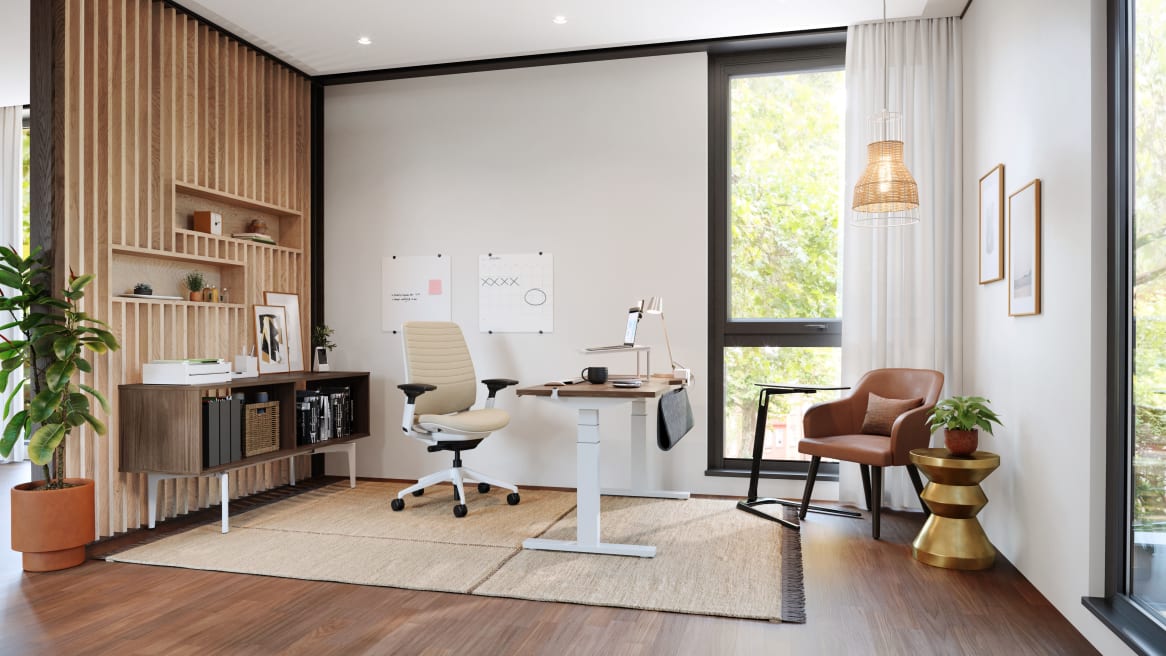The image depicts a well-organized, modern office space. At the center is a wooden table with a white frame, supported by two white legs. To its left stands an office chair characterized by a light green back, black armrests, black wheels, and a predominantly white structure with a black swivel base. Behind the chair is a feature wall, part wood and part white, with two pieces of paper attached to it—one featuring four black X's and an O, and the other a pink post-it note with adjacent black text. Adjacent to this, a section of untreated wood with two rectangular cut-outs serves as a unique shelving space housing small plants.

Beneath the shelving is a brown cabinet displaying pictures and a white printer. In the bottom left corner, an orange ceramic pot with a tall green plant featuring large leaves adds a touch of nature. On the right side of the room stands a brown leather armchair with a matching pillow, elevated on four wooden legs. Near it, a gold-colored table holds a ceramic planter with another green plant. Above the armchair, an orange light fixture hangs from the ceiling, casting a warm glow. Behind the armchair, a large floor-to-ceiling window framed in black and covered by white curtains allows natural light to filter in.

The right wall is adorned with two framed pictures with light brown wooden frames. The room's floor boasts a dark brown shade complemented by a centrally placed cream-colored carpet, enhancing the space's sophisticated ambiance.